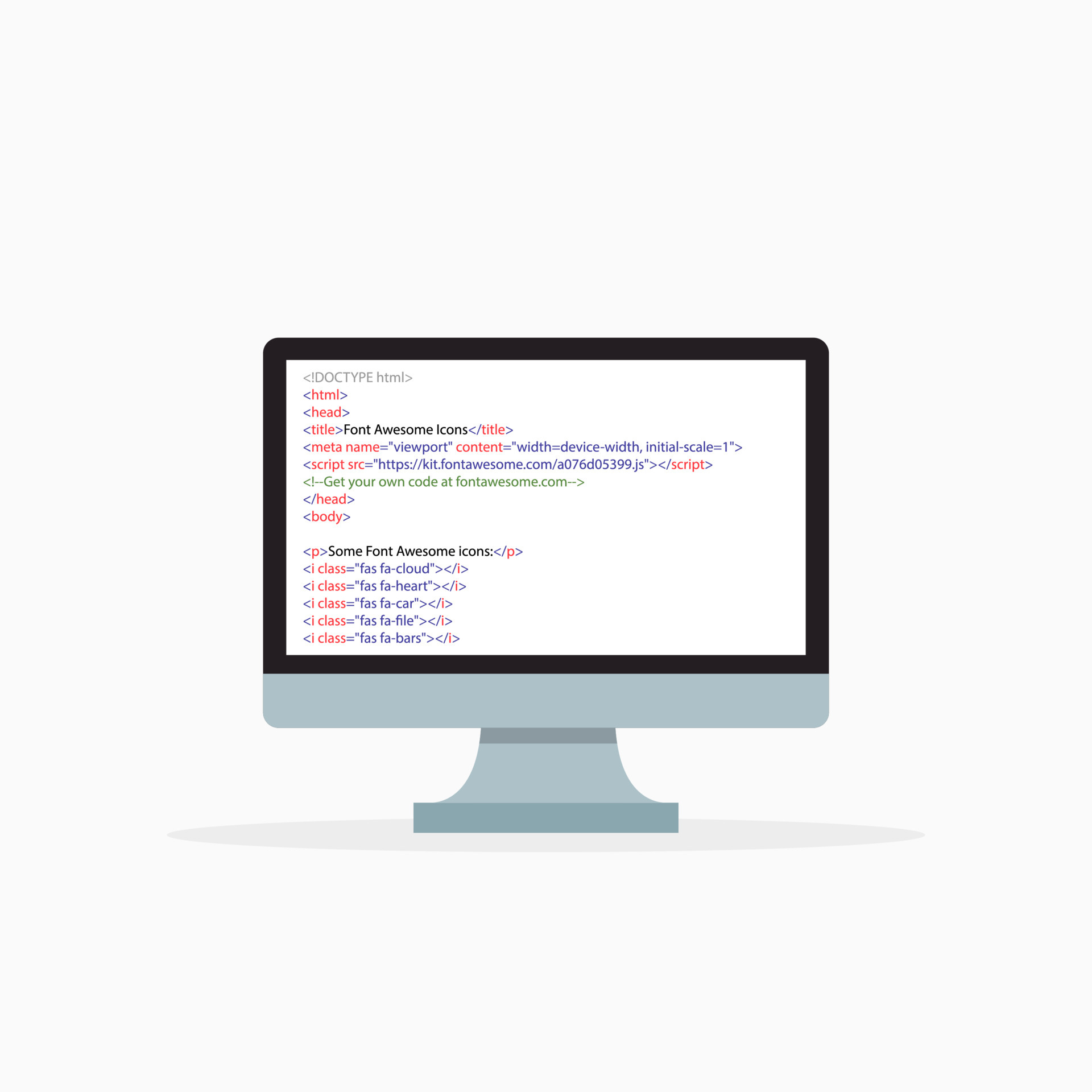The image depicts a cartoonish, digital rendering of a computer monitor against a white background. The monitor is outlined with a black frame and has a gray base. Displayed on the screen is a mixture of red, blue, black, and green text, representing various snippets of HTML and related coding languages. Notable elements of the code include: "DOCTYPE HTML" in red, "head," "title Font Awesome Icons /title" in various colors, and a meta tag detailing viewport settings. Additionally, there is a script reference to "https://kit.fontawesome.com/a076d05399.js" and a notation in green text stating "Get your own code at fortawesome.com." The screen is filled with these technical details, showcasing a colorful array of coding syntax.